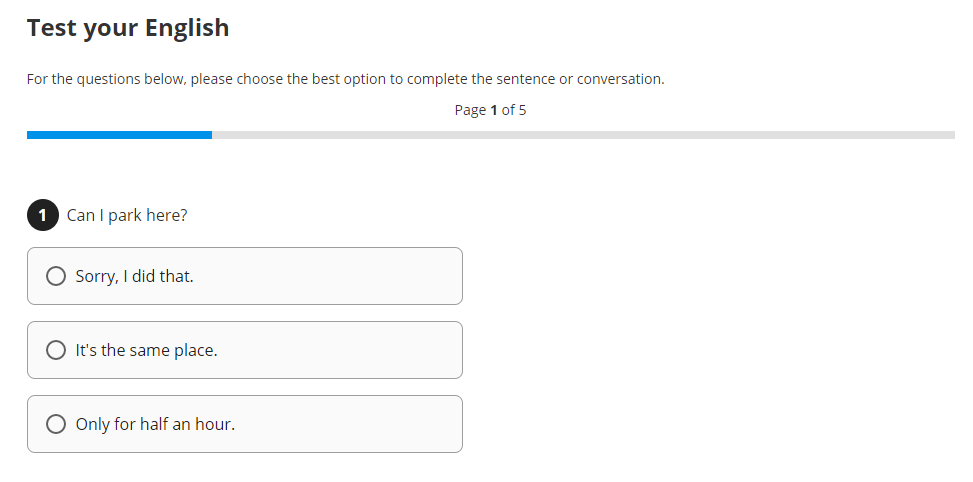This is a detailed description and cleaned-up caption for the image:

The webpage features an interactive English language assessment tool titled "Test Your English." The interface is minimalist, with a white background that highlights clarity and focus. At the top, a heading reads "Test Your English," followed by instructions that state: "For the questions below, please choose the best option to complete the sentence or conversation." 

Displayed prominently on the screen is the first question out of five, accompanied by a status bar that is approximately one-quarter filled in blue, indicating progress through the test. The sample question reads, "Can I park here?" Below this question are three multiple-choice responses: 

1. "Sorry, I did that."
2. "It's the same place."
3. "Only for a half hour."

Users are prompted to select one of these options as their answer. The design suggests functionality for testing one's proficiency in English, possibly for educational purposes or employment screening. The absence of additional graphics or distractions ensures that the user's focus remains solely on the task at hand.